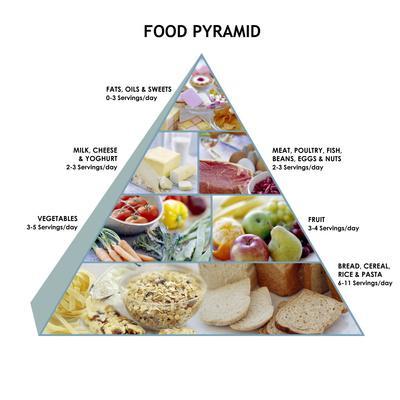This image features a detailed, somewhat 3D, depiction of the classic food pyramid against a completely white background. At the top, the black, all-caps text "FOOD PYRAMID" is positioned, taking up minimal space. Below this, a large, gray, triangular section dominates the image, with a light gray shadow hinting at the pyramid's 3D structure. Starting from the apex, the pyramid categorizes food groups with their corresponding servings per day and includes small photographic images for visual aid.

At the very top left, labeled "Fats, Oils, and Sweets," the section suggests 0-3 servings per day and displays blurry images of chips, pastries, and other sweets. Directly below this, the pyramid divides into two sections: to the left, "Milk, Cheese, and Yogurt," recommending 2-3 servings per day, illustrated with blocks of cheese and butter; to the right, "Meat, Poultry, Fish, Beans, Eggs, and Nuts," also advising 2-3 servings per day, depicted with images of eggs, raw meats, and beans.

Further down to the left, the segment for "Vegetables," suggesting 3-5 servings per day, features vibrant images of carrots, tomatoes, peppers, and other raw vegetables. Adjacent to this on the right, the "Fruits" section, recommending 3-4 servings per day, shows pictures of apples, oranges, grapes, pears, and bananas. 

Finally, at the base of the triangle, the largest section is labeled "Bread, Cereal, Rice, and Pasta," advising 6-11 servings per day, depicted with ample images of bread, cereal, and pasta, providing a strong foundation for the pyramid.